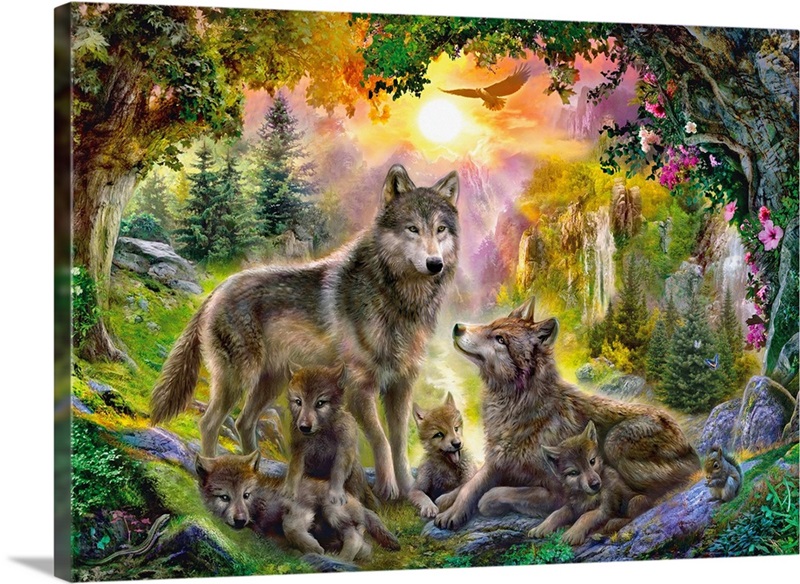The artwork is a vivid, colorful drawing of a natural outdoor scene featuring wolves, trees, and other wildlife elements. Dominating the center are two large wolves—one standing on the left, facing right, and one lying down on the right, appearing to look up at the standing wolf. Surrounding them are four smaller wolf cubs. In the lower right corner, a small squirrel is visible. The background is rich with nature, featuring trees adorned with pink and magenta flower petals, with particularly large trees situated in the top right and top left corners. The sun is centrally positioned, shining over distant mountains, accompanied by an eagle soaring nearby. The wolf lying down appears to be injured, marked with reddish-purple streaks.